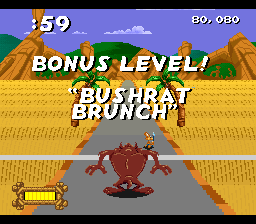The image depicts a screenshot from a video game. The top and bottom of the screen feature black borders framing the action. A clear blue sky adorned with fluffy white clouds stretches across the background. At the top of the screen, a timer counts down from 59 seconds alongside a score display showing 80,000 points in white text. Centered in the middle of the screen, bold white writing announces a "Bonus Level" titled "Bush Rat Brunch." Lush green mountains loom in the distant background, punctuated by imposing rock formations. Brown grass flanks the scene, with a narrow road cutting through the center. Distinguishing the road are contrasting stripes of gray and light gray. Dominating the foreground is a large, brown creature reminiscent of the Tasmanian Devil character, seen from behind. The creature has a broad back, small head, and disproportionately large hands and feet.